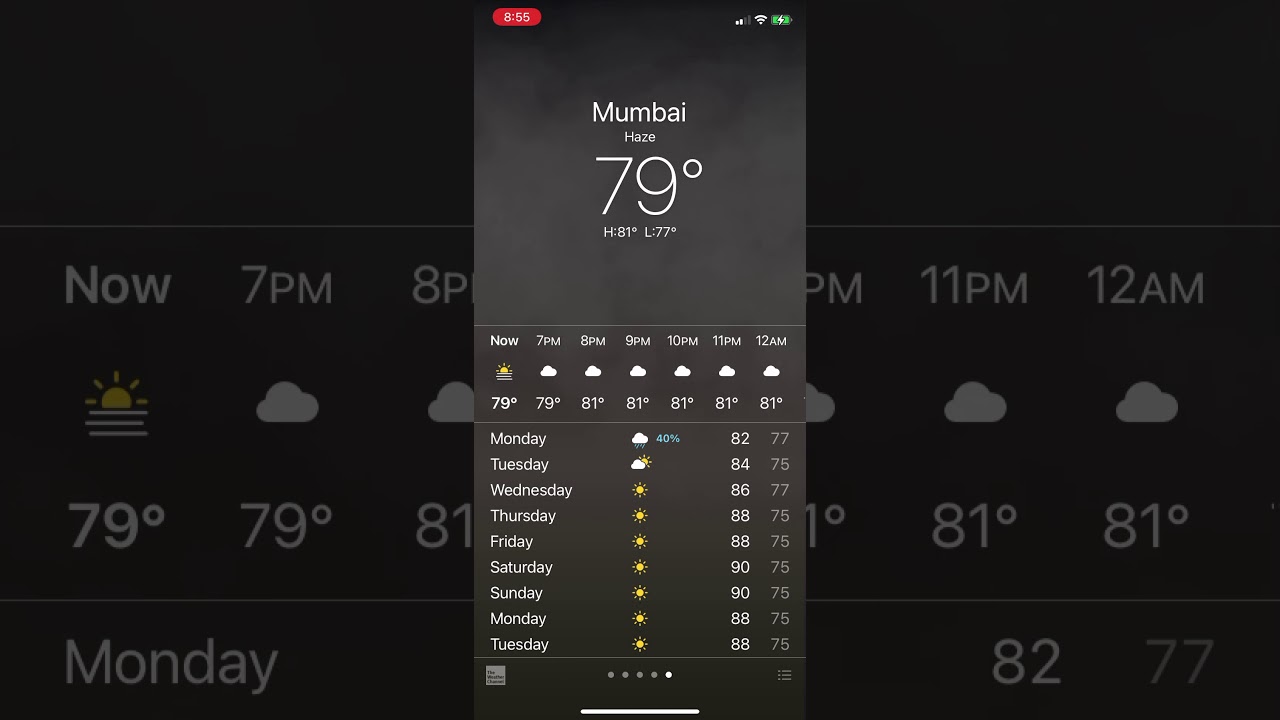This is a detailed screenshot of a weather app on a smartphone, displaying the current and forecasted weather for Mumbai. The background prominently features the weather forecast for Monday, though the remaining days of the week are partially obscured. At the top of the screen, the app indicates the current condition with the word "Now," accompanied by a sun icon with three rays and a temperature reading of 79°F. The hourly forecast for Monday is also shown, starting with 79°F and rising slightly to 81°F by 12 AM.

In the top-left corner of the screen, a red oval icon displays the number 855. To the top-right, several status icons are visible, including a partially filled phone signal, a fully filled Wi-Fi signal, and a fully charged battery icon. In the middle section of the app, the location is clearly labeled as "Mumbai," with the current weather condition described as "Haze." The main weather readout also prominently displays 79°F, with a high of 81°F and a low of 77°F for the day.

Beneath the main temperature display, the detailed hourly forecast for the rest of Monday is shown, with each hour accompanied by a representative weather icon, transitioning from sunny at the current hour to cloudy in later hours. Below this, the app provides a brief weekly forecast, showing the progression from the current Monday to the following Monday and Tuesday, with corresponding weather icons and temperatures listed to the right of each day.